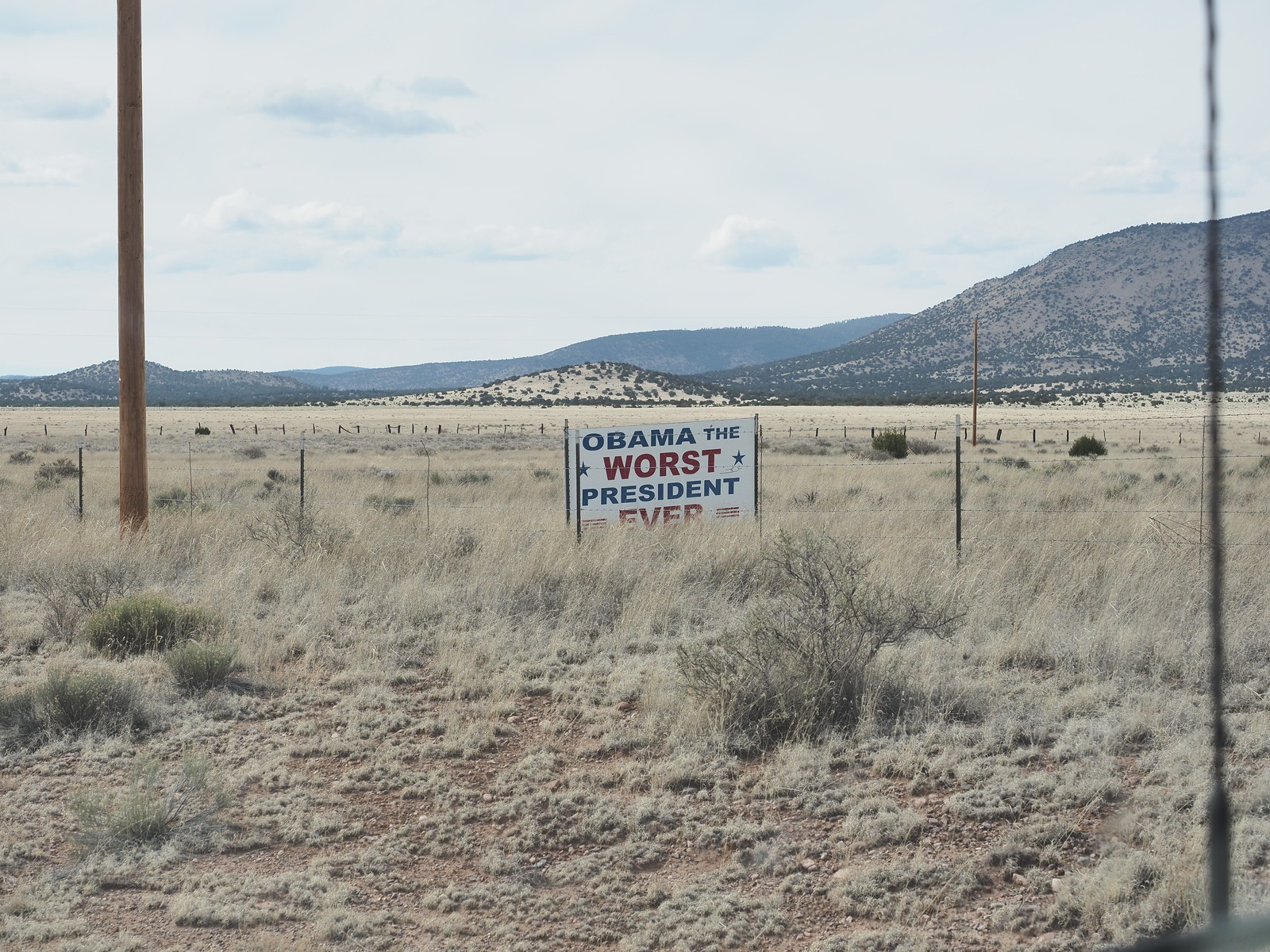A breathtaking desert landscape, reminiscent of scenes from classic Westerns, is marred by an incongruous political sign declaring "Obama, the worst president ever." The natural beauty of the area, characterized by rugged brush and majestic hills, is stunning, especially under the light of a setting sun. However, this serene vista is disrupted by the intrusive sign, which injects unnecessary political discourse into an otherwise pristine environment. The juxtaposition of the untouched wilderness and the abrasive political message exemplifies a rather thoughtless placement, detracting from the visual and emotional impact of the landscape. One can't help but imagine that any passerby with an appreciation for the scenery might feel compelled to remove the sign, restoring the view to its unblemished state.